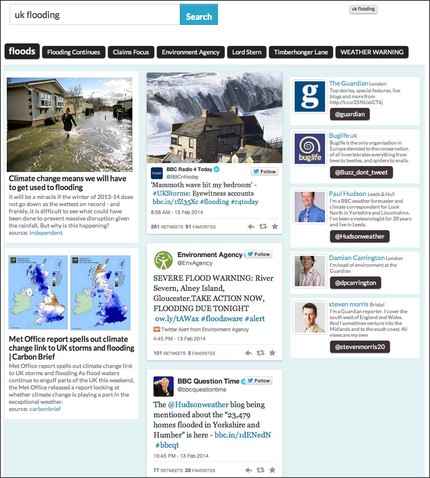The screen displays a webpage with various sections related to UK flooding and climate change. At the top, a blue-highlighted search bar reads "UK flooding." Below, a headline states "Flooding Continues: Claims Focus on Environment Agencies." Additional text mentions specific locations like Lord Stem, Timber Hogger Lane, and issues a weather warning.

A subheading warns that "Climate change means we'll have to get used to flooding." An image depicts a person walking through daytime floodwaters with visible sunlight. Another section describes an eyewitness account: "Mammoth wave hit my bedroom" and features a photo of waves crashing into a house.

Further text explicitly links climate change to UK storms and flooding, citing a Met Office report shared by Carbon Brief. An embedded Twitter follow button is positioned near information from the emergency agency, which includes a "Severe Flood Warning" for River Severn in Gloucester, advising immediate action for anticipated flooding tonight.

Lastly, BBC's Question Time and the Hudson Weather Blog mention the flooding of 23,479 homes in Yorkshire and Humber.